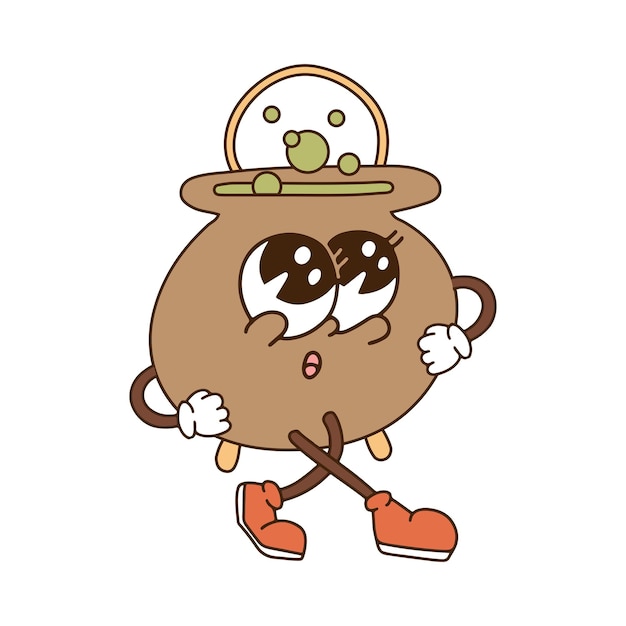This is a detailed, cartoon-like sketch of a whimsical character that resembles a pot or planter. The character features a light brown, circular body with a cylindrical head, which has an opening at the top. From this opening, green circular bubbles appear to be either entering or emerging. The character sports exaggerated black and white eyes, tiny pink lips, and an orange halo behind its head. It has dark brown limbs consisting of arms, which are bent and end in white gloves, and skinny, bendable legs. The legs terminate in pink or orange sneakers with white soles. Additionally, two orange pieces stick out from behind its back. The character is set against a white background, suggesting it is walking or dancing with one foot in front of the other and hands placed on its hips, looking up at the sky.